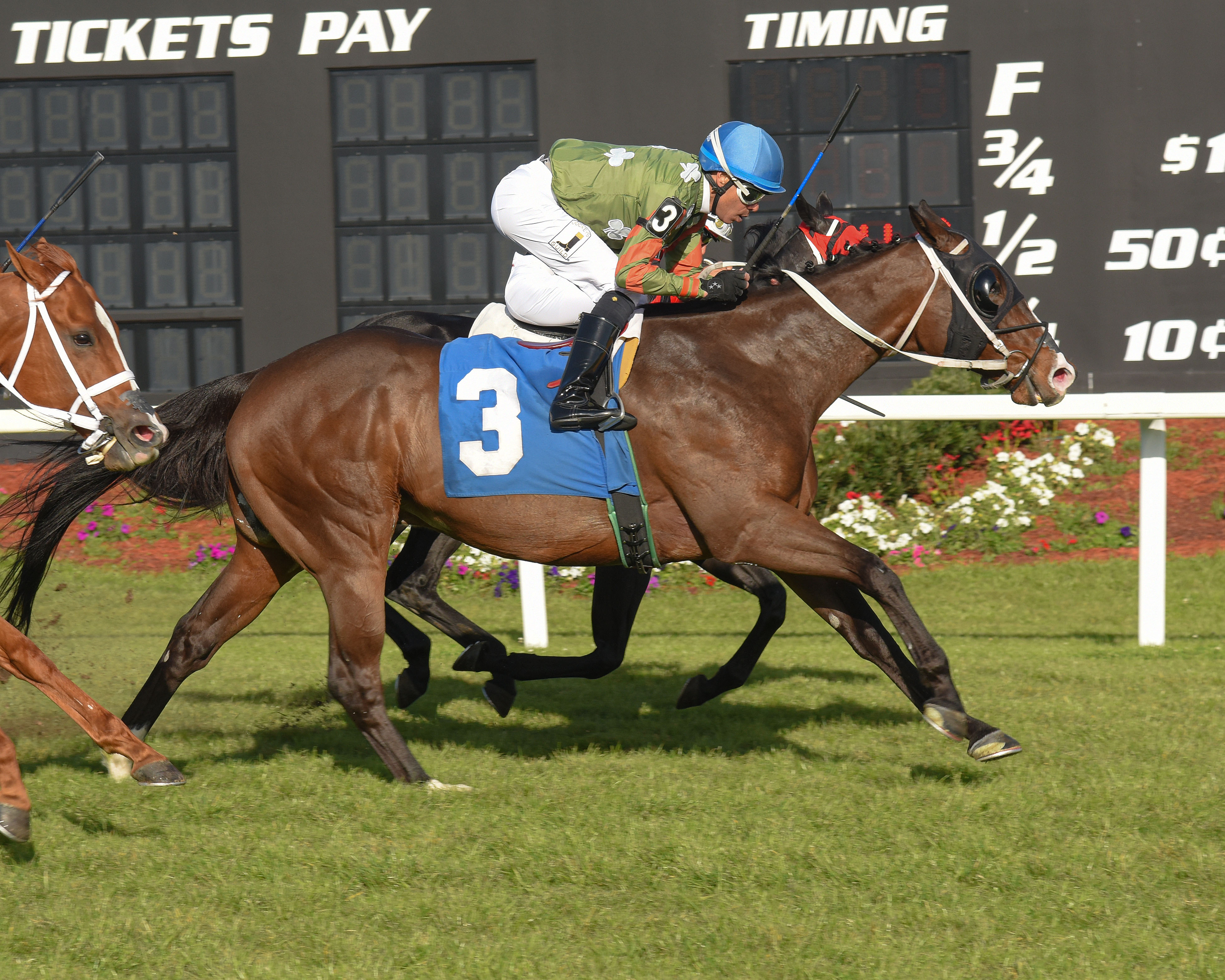In this dynamic outdoor horse racing photo, the focus is on a brown horse with dark brown legs and a black face covering. The horse is racing on a green grass track and bears the number three, highlighted on a blue flag strapped around its body. The jockey atop the horse is leaning forward, wearing white pants, black knee-high boots, and a long green shirt with distinctive orange stripes on the sleeves. He dons a blue helmet with white goggles, black gloves, and is clutching a black and blue whip. Behind this lead horse, another horse with a brown head and legs adorned with white straps is visible. In the background, a white fence runs in front of a large black scoreboard displaying "tickets pay" and timing details, contributing to the competitive atmosphere of the race.